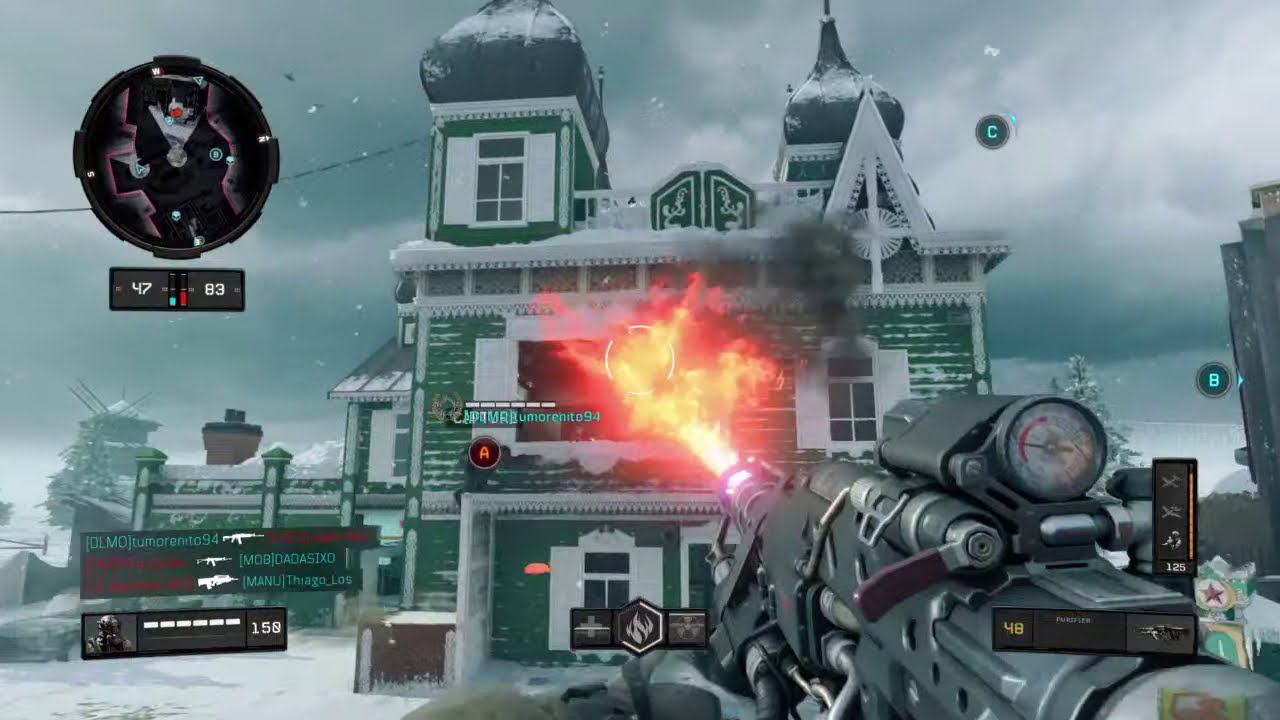The image is a detailed screenshot from a first-person shooter video game set in a snowy warscape. Dark gray clouds filled with small snow flurries dominate the background. In the foreground, a large green, three-story building with white shutters and a steeple is prominently targeted. The top left corner of the image shows the first-person view through a gun scope, with a red dot precisely sighted on another character’s forehead. Meanwhile, the bottom left corner displays gamer tags in red and light blue, alongside a full health bar. On the right side, a large, gray flamethrower with purple levers, gauges, valves, and a bright flame is positioned. The building appears to be under attack, with flames engulfing it and smoke rising, suggesting a deliberate attempt to burn it down. The building, which could be a home or a hideout, has an all-green facade with a triangular roof on the right and a gray-roofed tower on the left. Stats related to the game are also visible in the lower right corner, indicating the number of players killed.